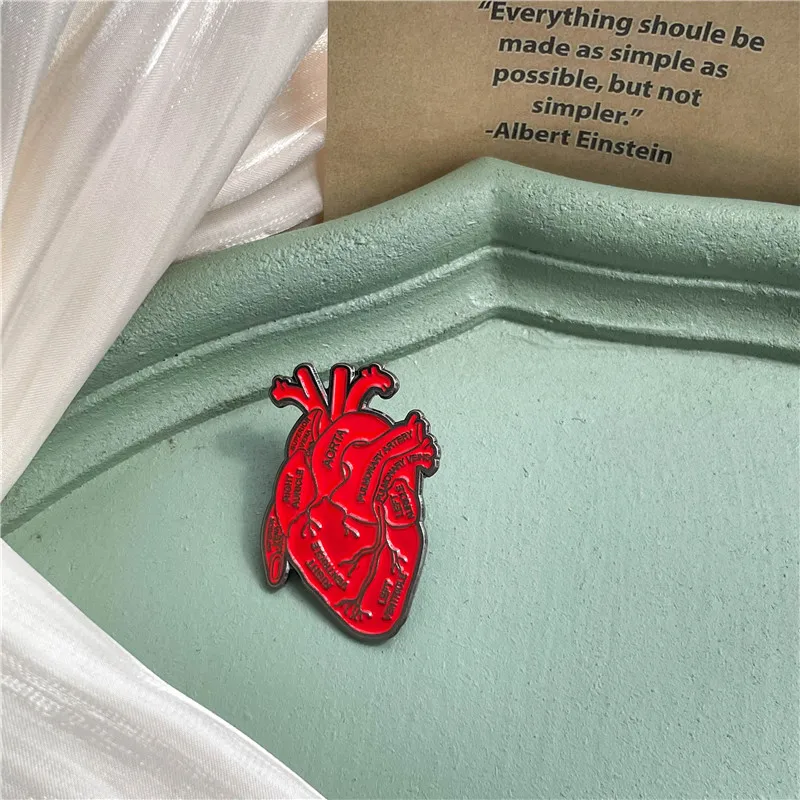This image features a deep crimson, heart-shaped metal pin, intricately designed to resemble a human heart organ with labeled sections. Detailed labels include aorta, pulmonary artery, pulmonary veins, left ventricle, and right ventricle, each clearly marked in black. The pin has a black outline and rests on a muted light green wood tray. A piece of white plastic is wrapped around the left corner of the tray, adding another layer of texture to the scene. In the upper right corner, a brown paper bag with blue text displays an Albert Einstein quote: "Everything should be made as simple as possible, but not simpler." The background varies in description but suggests a mixture of teal and tan hues, contributing to the overall photorealistic quality of the image.